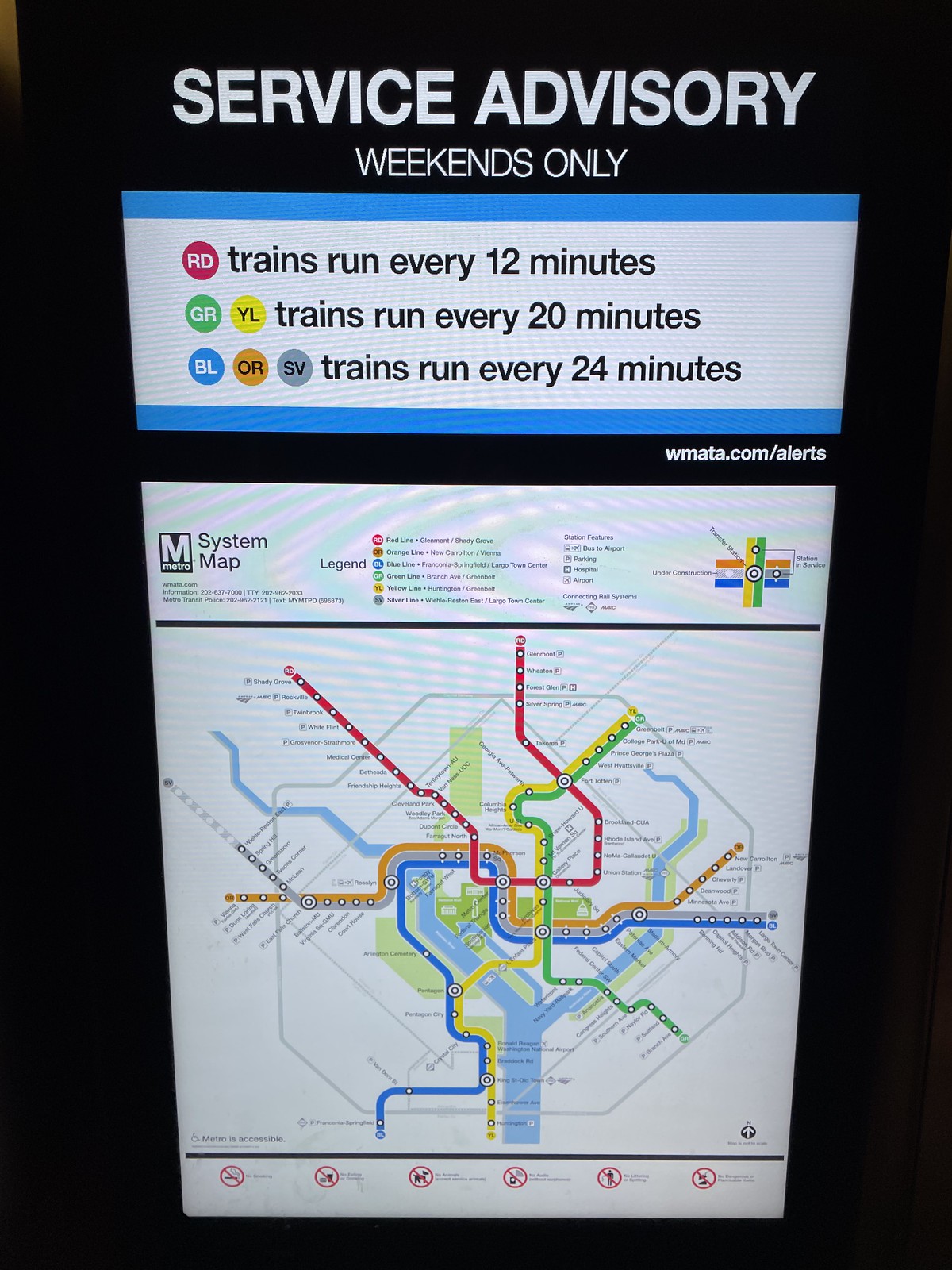This image depicts a rectangular digital display typically found in a metro station, featuring a comprehensive service advisory. The sign's black frame encloses information about weekend train schedules, displayed in bold white text at the top reading, "Service Advisory, Weekends Only." Directly beneath this, a horizontal rectangle with blue headers and footers against a gray background provides train frequencies: a red circle labeled "RD" indicates trains run every 12 minutes; green "GR" and yellow "YL" circles stating trains run every 20 minutes; and blue "BL," orange "OR," and silver "SV" circles showing trains run every 24 minutes. This section is anchored by the URL "wmata.com/alerts" in white text at the lower right.

Below this advisory, a slightly tilted, elongated system map occupies the bottom portion of the display. This gray-background map features color-coded lines representing different metro routes, labeled in a legend at the top: red, green, yellow, blue, orange, and silver lines. The map details all stops along each route. At the bottom, icons in red circles indicate prohibited activities, such as no smoking, no pets, no food or drinks, and no littering.